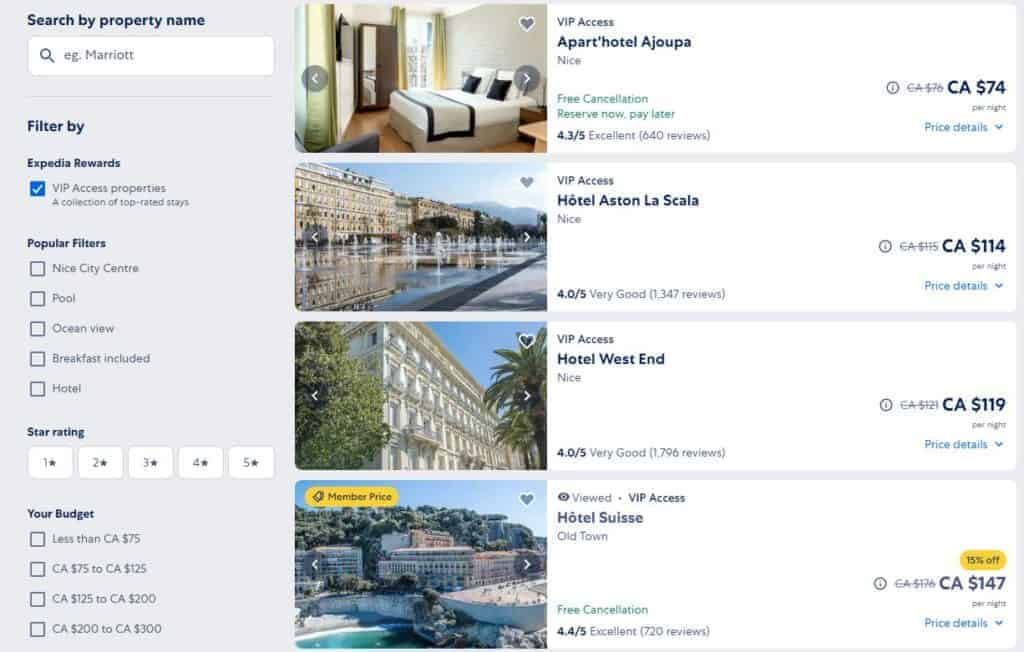Screenshot from a hotel booking website, showcasing a user interface with various search filters and property listings. On the left side, a vertical grey column extends significantly into the page, containing numerous filter options, including checkboxes for amenities such as "City Center," "Pool," "Ocean View," and "Breakfast Included." Below these are additional filters for star ratings and budget preferences.

The central and right portions of the page feature a vertically arranged list of property images. Each property is displayed in a horizontal listing format, with a photo of the accommodation on the left, followed by its name. To the right of each photo, the cost per stay is prominently displayed, with blue text reading "price details" located just below the price. The overall background of the page is white, creating a clean and organized look, while the detailed filters remain easily accessible within the grey sidebar.